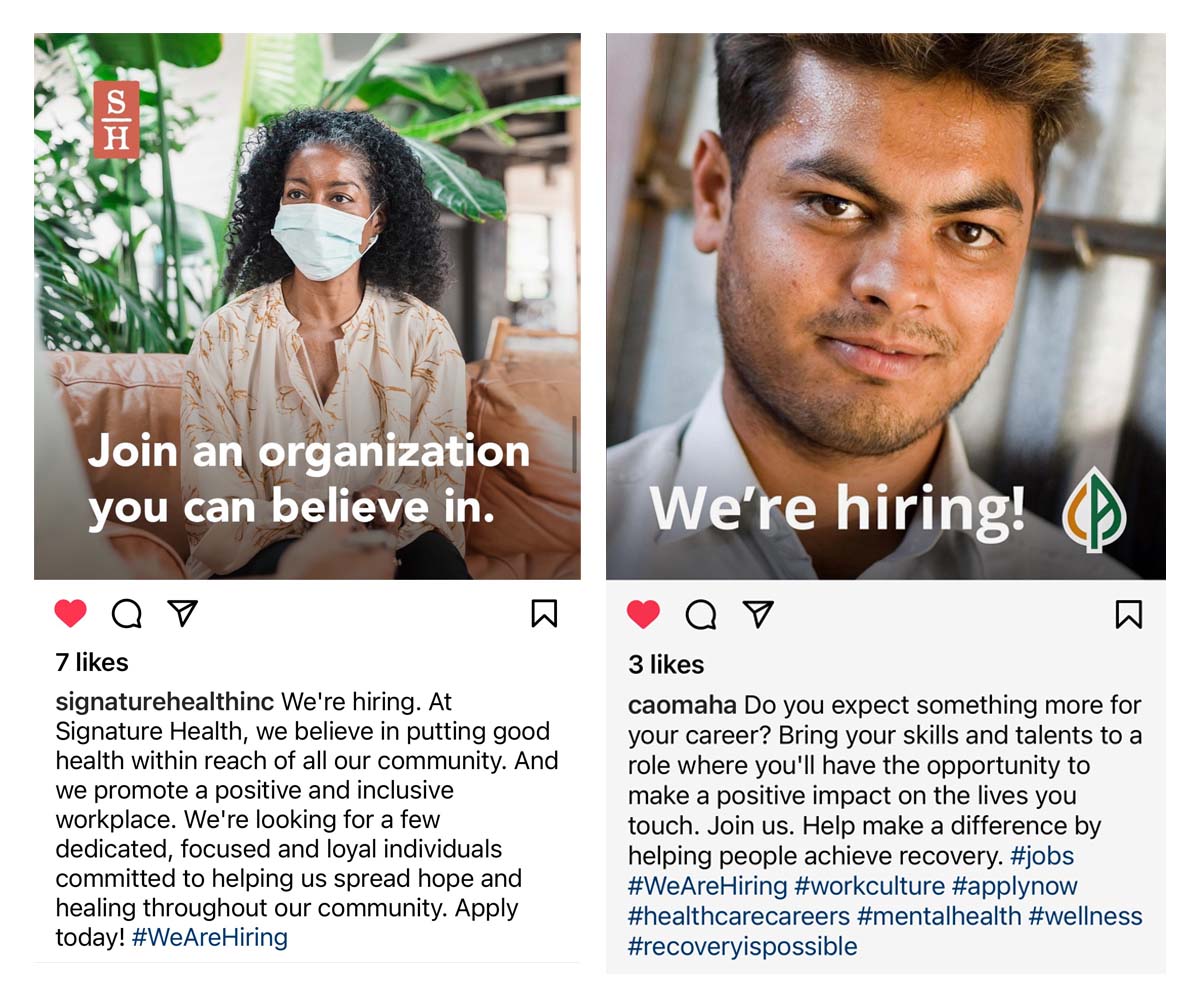**Detailed Caption:**

This image is a screenshot of a social media post advertising job openings for two organizations. The layout is split into two sections: the left side and the right side, each featuring a different individual and message.

On the left side of the image, there is a photograph of a woman with black hair, wearing a dress shirt in shades of brown. Her face is partially obscured by a mask, and she is seated on a couch. Superimposed on her picture is the text, "Join an organization you can believe in," written in white lettering. The screenshot shows that the original poster liked this image, indicated by the dark red heart icon, and it has received a total of seven likes. This segment is branded with the name "Signature Health Inc."

On the right side, there is a photograph of a man with short brown hair, dressed in a white dress shirt. He has a self-assured expression, with slightly raised eyebrows, and is looking directly at the camera. This image bears the text, "We're hiring," also in white. It features a distinctive leaf logo, split with the left half in red and the middle and right sides in dark green. This post, attributed to an organization named "Kaomaha," is similarly liked by the same user, as shown by the dark red heart icon, and it has garnered three likes.

Both sections of the post aim to attract potential job applicants, with thoughtful and visually engaging presentations from their respective organizations.